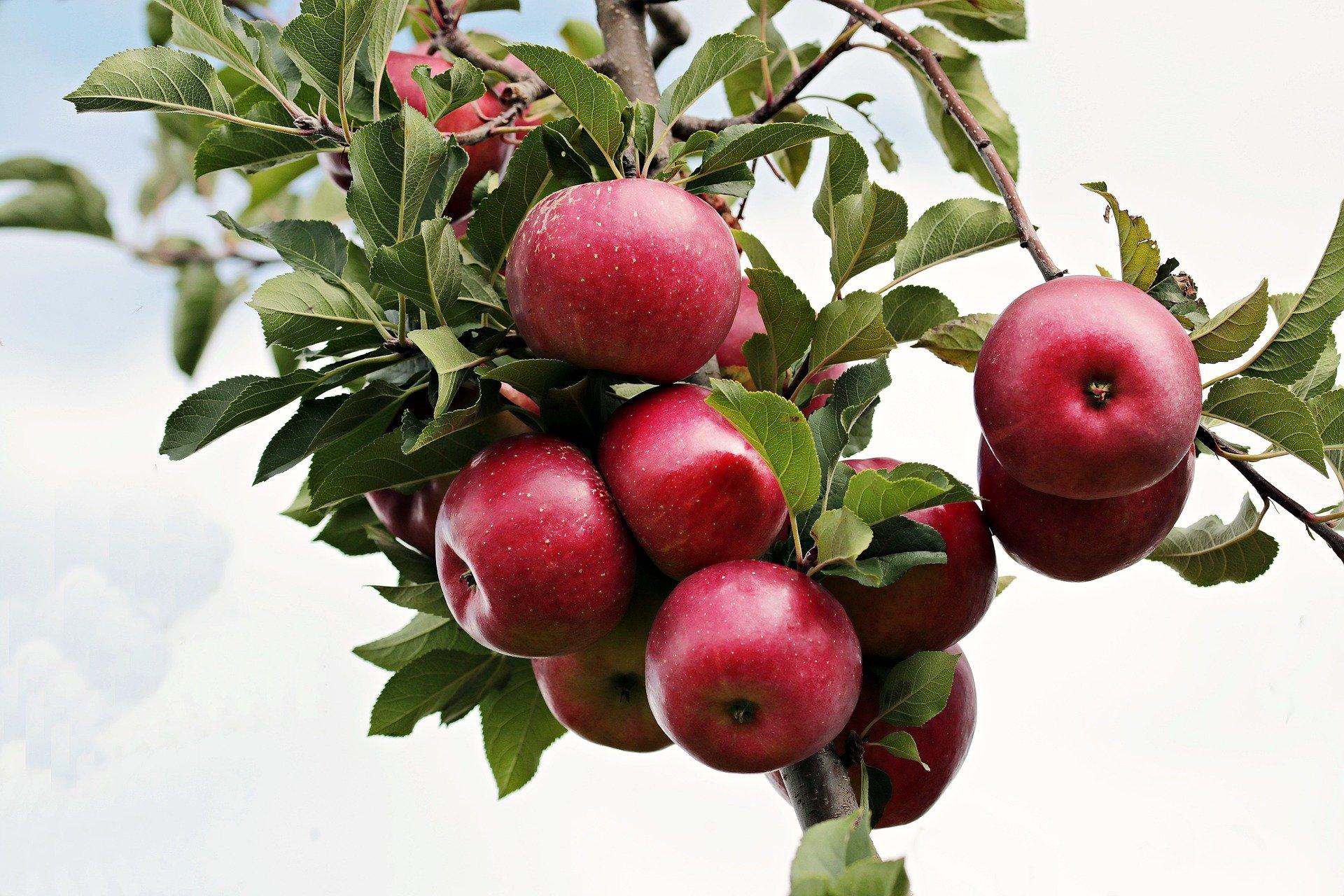In this vibrant daytime photo taken in a garden, we see a close-up view of a hanging branch from an apple tree. The branch is adorned with lush green leaves and features a prominent cluster of about six or seven ripe, red apples. The apples look fresh and ready to be picked, with a few showing tiny white spots, but are largely clean and glistening in the sunlight. The healthy appearance of both the apples and the tree suggests an optimal growing environment. The background captures a partly washed-out blue sky with white clouds, emphasizing the brightness of the scene. Some apples are tucked behind leaves, adding a sense of depth and abundance to the image.